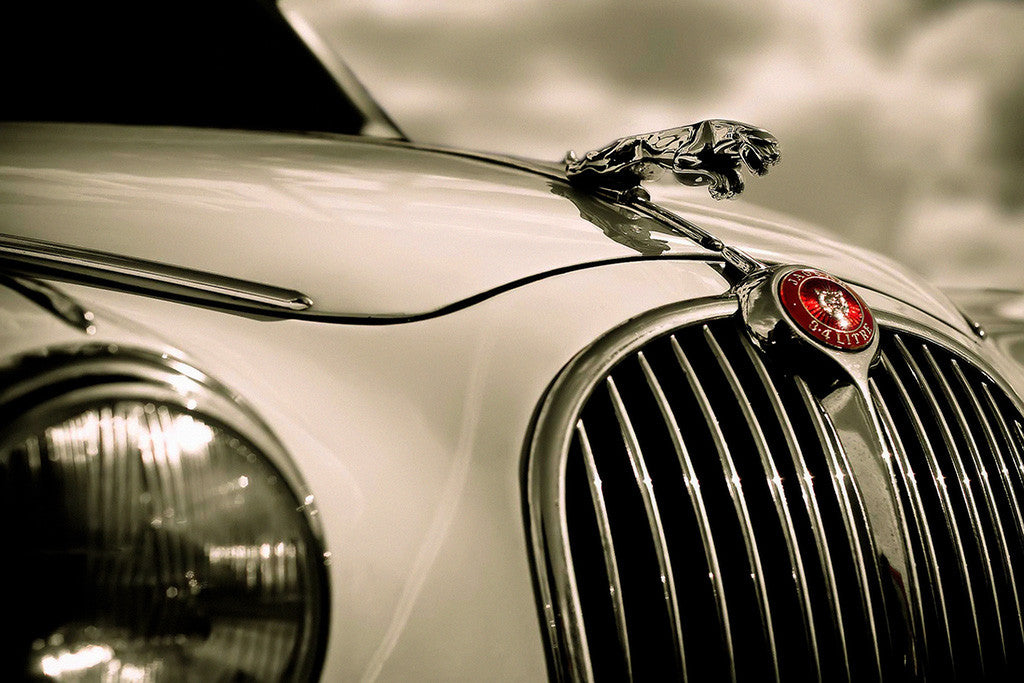The image showcases a luxurious Jaguar car, meticulously capturing its distinctive features. Dominating the center is the iconic Jaguar emblem, prominently displayed on the front hood. The windshield is positioned in the top left corner, while the right headlight occupies the bottom left. Adjacent to the headlight in the bottom right is the car’s polished grill, adorned with the text "Jaguar 3.4 liter" above it. The car’s sleek hood stretches to the left of the emblem, and the background in the top right corner features a blurred, gray sky, hinting at an outdoor daylight setting. The car's elegant color palette includes shades of red, silver, gray, black, and a touch of white, enhancing its sophisticated appearance. The photo is taken at an angle, emphasizing the front part of the car and capturing the essence of its design.